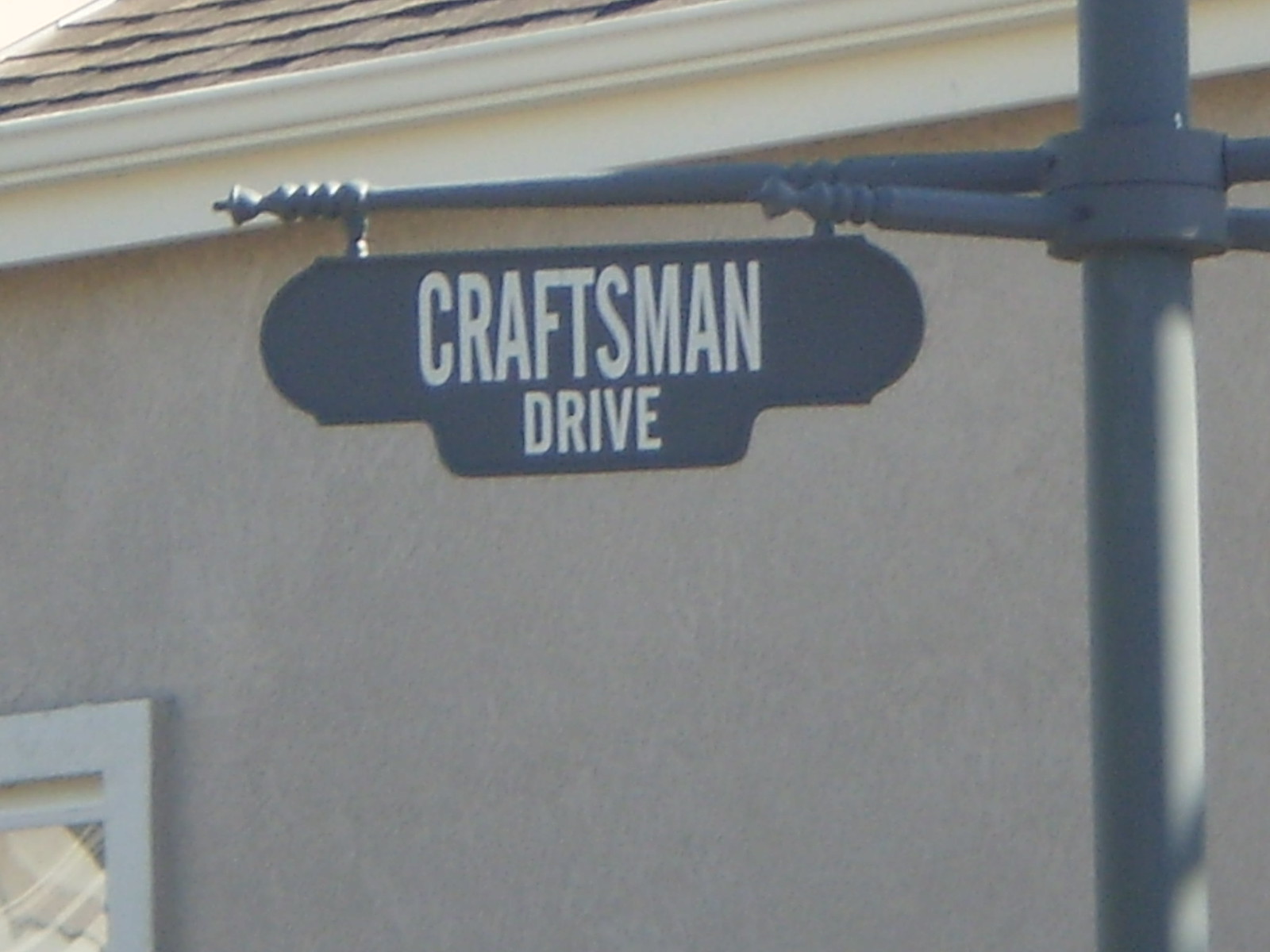In this daytime photograph, the focal point is a gray street sign mounted on a smoke-gray metal pole, which extends vertically through the image. The sign has a classic, clean design with white lettering that reads "Craftsman Drive." To the right of the sign, partially visible, is a smaller metal rod extending horizontally. In the background, a tan stucco house with white trim surrounds a partially visible window in the bottom-left corner. The house features a brown-tiled roof and tan roof border, catching sunlight that highlights the texture and details of the materials. The photograph captures a sunny, well-lit day, adding a warm glow to the overall scene.